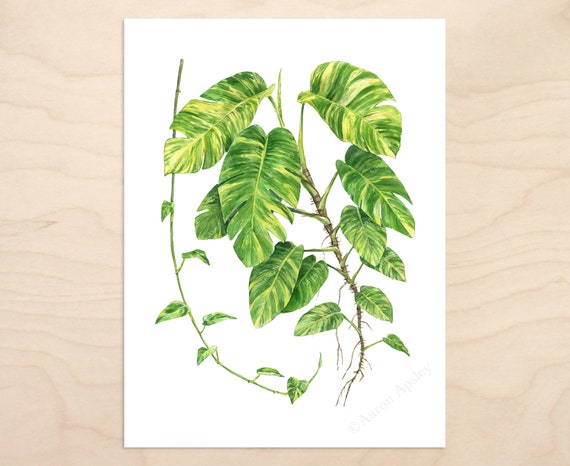This is a detailed image of a drawing depicting a vine with various green leaves, laid flat on a white piece of paper. The paper rests on a light tan wooden table. The vine in the center of the drawing features leaves that range in size, with smaller leaves at the root and progressively larger ones toward the top. These leaves exhibit various shades of green, intermixed with some yellow, and occasional brown spots. On the left side of the drawing, there's a separate, smaller vine adorned with tiny green leaves. The overall color palette of the image is quite basic, featuring shades of green, yellow, tan, and brown. Some parts of the main vine's leaves appear slightly split, adding texture to the illustration.